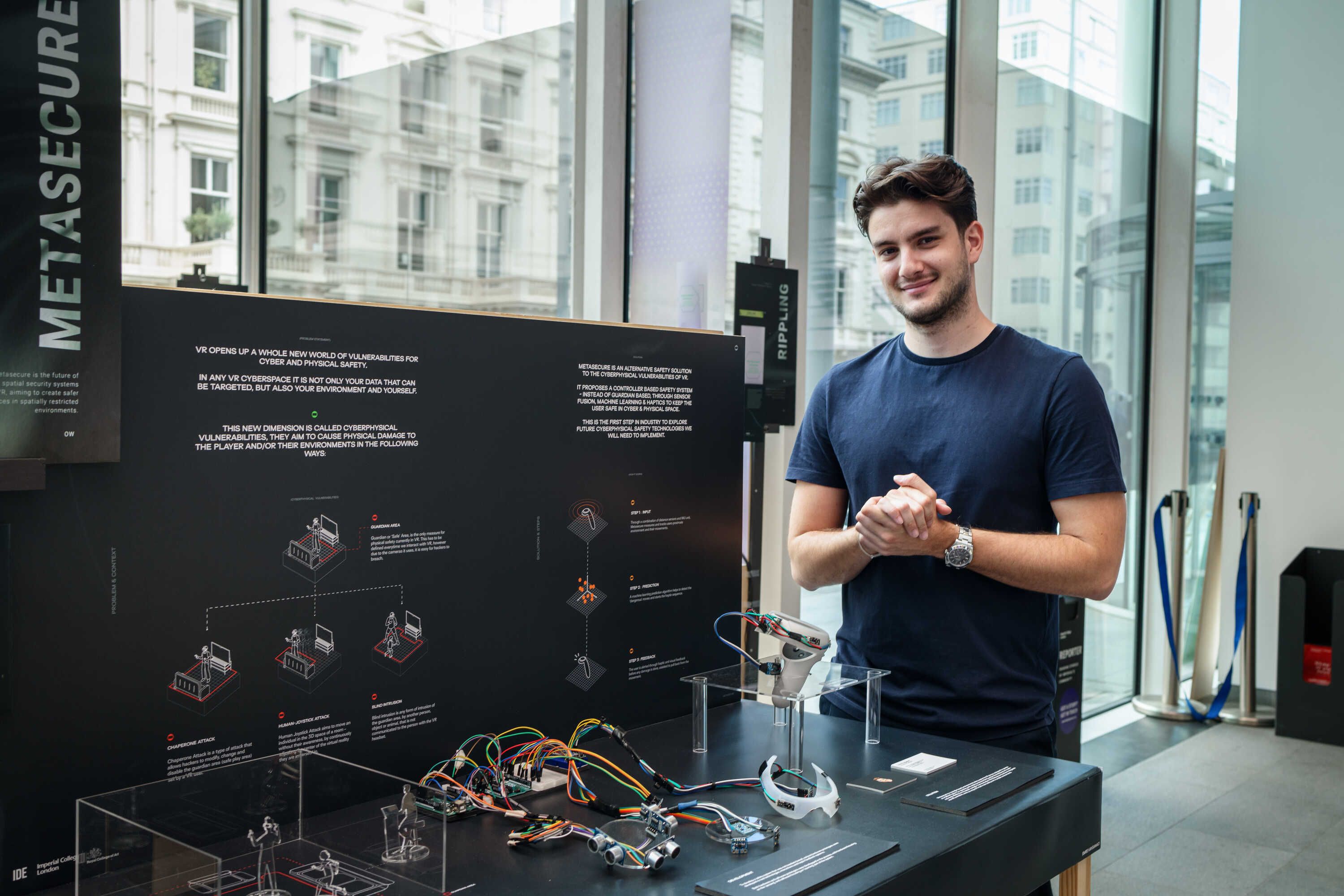The photograph captures the interior of an office building lobby, identified by its modern design and floor-to-ceiling glass windows that offer a clear view of the well-preserved, light-colored brick and stone buildings outside, likely from the turn of the century. It is daytime in a business district. The focal point is a young man, appearing to be in his late 20s or early 30s, with brown hair, a light beard, and a medium build, typical of European descent. He is wearing a blue short-sleeved t-shirt and a wristwatch on his left wrist, standing confidently with his hands clasped together, smiling. The man is presenting an invention displayed on a dark-colored table, which features various acrylic stands, white plastic components, and brightly colored wires, suggestive of a computer engineering project. Behind the table, a professionally done black poster board labeled "Meta-Secure" provides detailed explanations and diagrams of his invention. The concrete floor and the light streaming through the large windows frame the scene, enhancing the professional and innovative atmosphere of the setting.